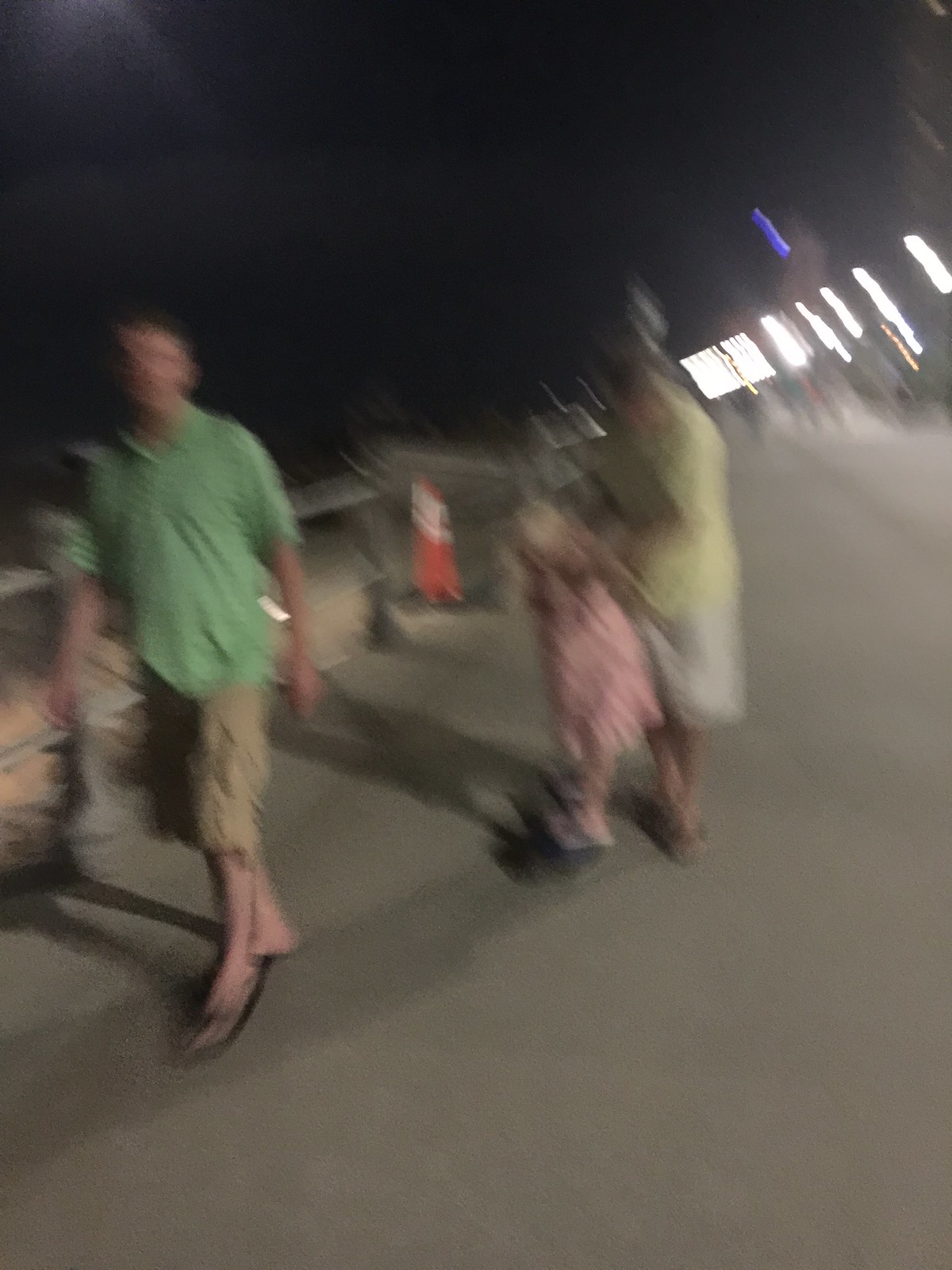In a dimly lit outdoor setting, three figures – two adults and a child – walk single file along what appears to be a boardwalk that slopes downward, possibly towards a beach. A blurred orange object, likely a traffic cone with a white top, marks a cautionary point, suggesting restricted access. Leading the group is a man donning a green button-down short-sleeve shirt, khaki cargo pants, and flip-flops. His dark hair merges with the night sky, making it difficult to distinguish. Following him is a small girl clad in a pink dress and black flip-flops, though her feet appear blurry. Trailing behind is a woman, dressed in a yellow top and a white garment that could be either a skirt or baggy pants. In the upper right corner, bright, blown-out white bars – possibly from a stationary light source captured with camera movement – dominate the scene, adding an ethereal quality to the photograph.